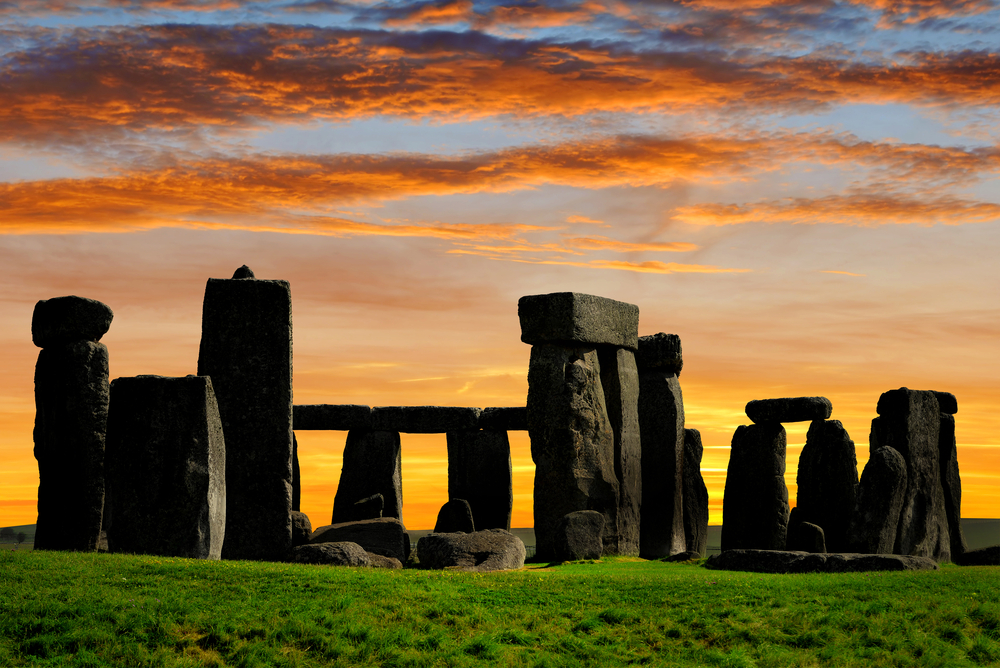A captivating photograph of Stonehenge set against a stunning sunrise. The ancient, gray and dark stones stand tall on a lush, green grassy field. From this side view, most of the rectangular stones are visible, including those that form the iconic lintel structure, with additional smaller stones scattered around. The sky above transitions dramatically from deep blues at the top to vibrant oranges, auburn, and yellows closer to the horizon, streaked with lines of clouds. The lighting creates a striking silhouette effect, highlighting Stonehenge against the warm glow of the rising sun, with intricate details of the stones' cracks and crevices faintly visible.